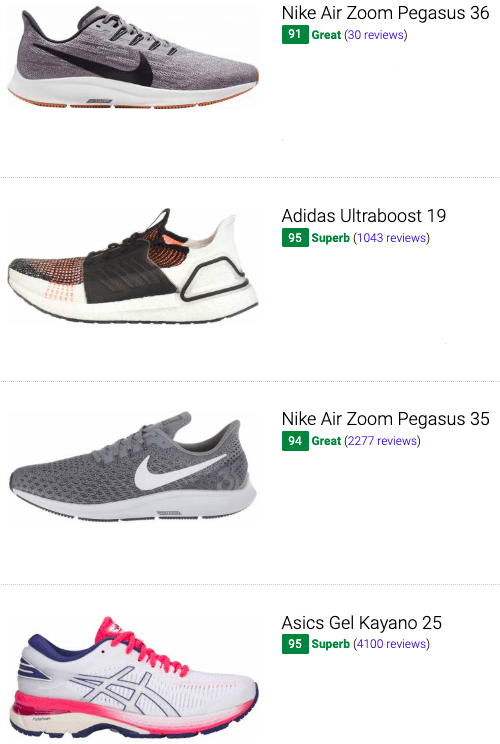This is a detailed screenshot from an undisclosed webpage showcasing several pairs of shoes available for sale. 

1. The first shoe, a gray Nike Air Zoom Pegasus 36, is oriented to the right. It features a black Nike swoosh on the side, with a white midsole and beige-colored treads on the very bottom. The corresponding text to the right indicates it has a rating of 91 based on 30 reviews.

2. The second shoe, an Adidas Ultra Boost 19, faces the left. It has a white body with a black mesh upper area overlaying an orange base around the tongue. The rear and bottom parts of the shoe are white. To the right, the text notes an impressive rating of 95, classified as superb, derived from 1,043 reviews.

3. The third shoe, another Nike model, is the Air Zoom Pegasus 35. This shoe also faces the left and is gray in color. It features a white Nike swoosh on the side, gray laces, and a white midsole. The text highlights a high rating of 94, described as great, with feedback from 2,277 reviews.

4. The final shoe in the screenshot is the Asics Gel Kayano 25, directed to the right. This predominantly white shoe features a black outlined design on the side, bright pink laces, and a bright pink section that extends towards the front. The midsole is white with some pink accents. The text indicates an exceptional rating of 95, termed superb, from 4,100 reviews.